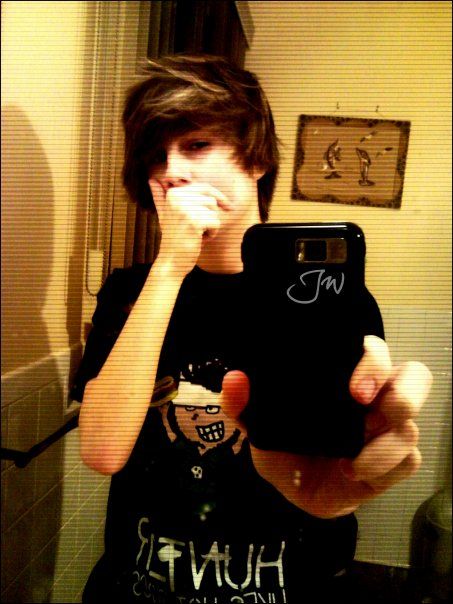A young teenage boy with an emo style is taking a selfie in a bathroom mirror using a mobile phone with a plain black case that has "JW" written on it. He has long, shaggy hair swooping to the left and is wearing a black t-shirt featuring a cartoon character with dark hair and a large smile, holding a hot dog. The text on the shirt appears to say "Hunter," although it’s seen backward in the reflection. The boy has his right hand over his mouth, creating a cool, mysterious look. The background includes tiled walls and possibly window blinds with a muted, yellowish filter adding a vintage feel to the photograph. There’s also a picture hanging on the wall behind him, contributing to the setting's casual, indoor ambiance.